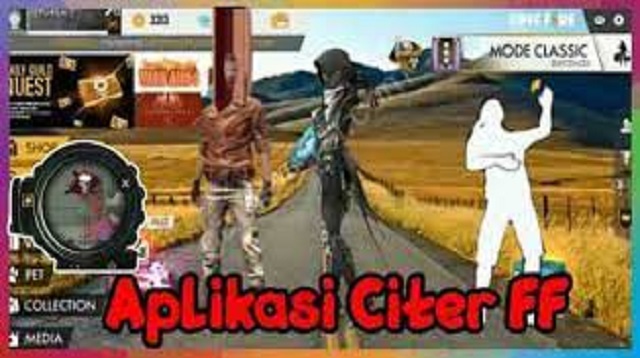This blurry rectangular image, horizontally aligned, features a vibrant multicolored border. Starting at the top left and moving clockwise, the border transitions through various colors: purple to gray to yellow to pink to purple along the top, purple to green to blue down the right side, blue to orange to red to dark pink along the bottom, and dark pink to purple to blue up the left side.

Inside this colorful frame, the scene depicts a road flanked by fields of brown grass, with mountains in the background under a blue sky. Central to the image are three indistinct game characters. The character on the left wears a brown or gold shirt and silver pants. The middle figure appears non-human and is dressed in a black uniform, perhaps with a black mask and black pants complemented by silver on top. The character on the right is represented as a white silhouette, lacking detailed features. 

At the top of the image, there is a sign reading "Mode Classic," indicating a game mode. Below, in bold red letters outlined in black, the text reads "APLIKASI CITER FF."